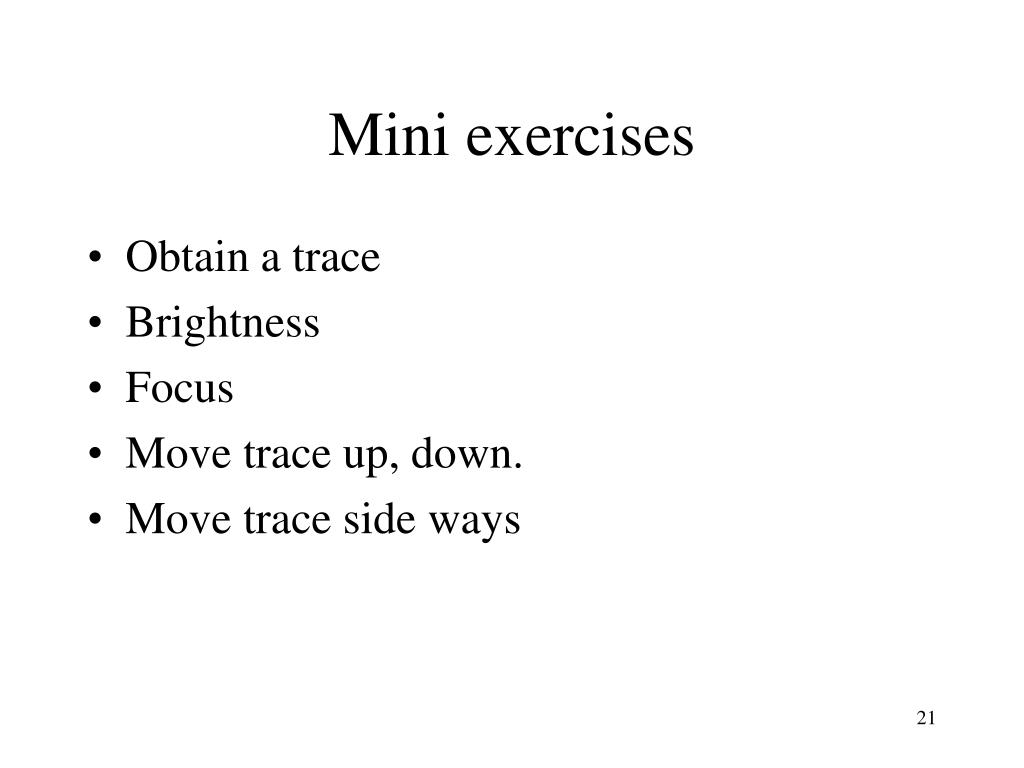The image appears to be a slide from a presentation or part of a lesson plan with a simple and straightforward design. It features a clean white background with black text in Times New Roman font. At the top, centered horizontally, is the title "Mini exercises," with 'Mini' capitalized and 'exercises' in lowercase. Below the title, there are five bullet points arranged in a vertical list, each preceded by a small black circular bullet. The bullet points read as follows: 

1. Obtain a trace
2. Brightness
3. Focus
4. Move trace up, down
5. Move trace sideways

Additionally, in the far right corner, there is a small, black number "21." The overall appearance of the slide is minimalistic, emphasizing clarity and simplicity in conveying information.